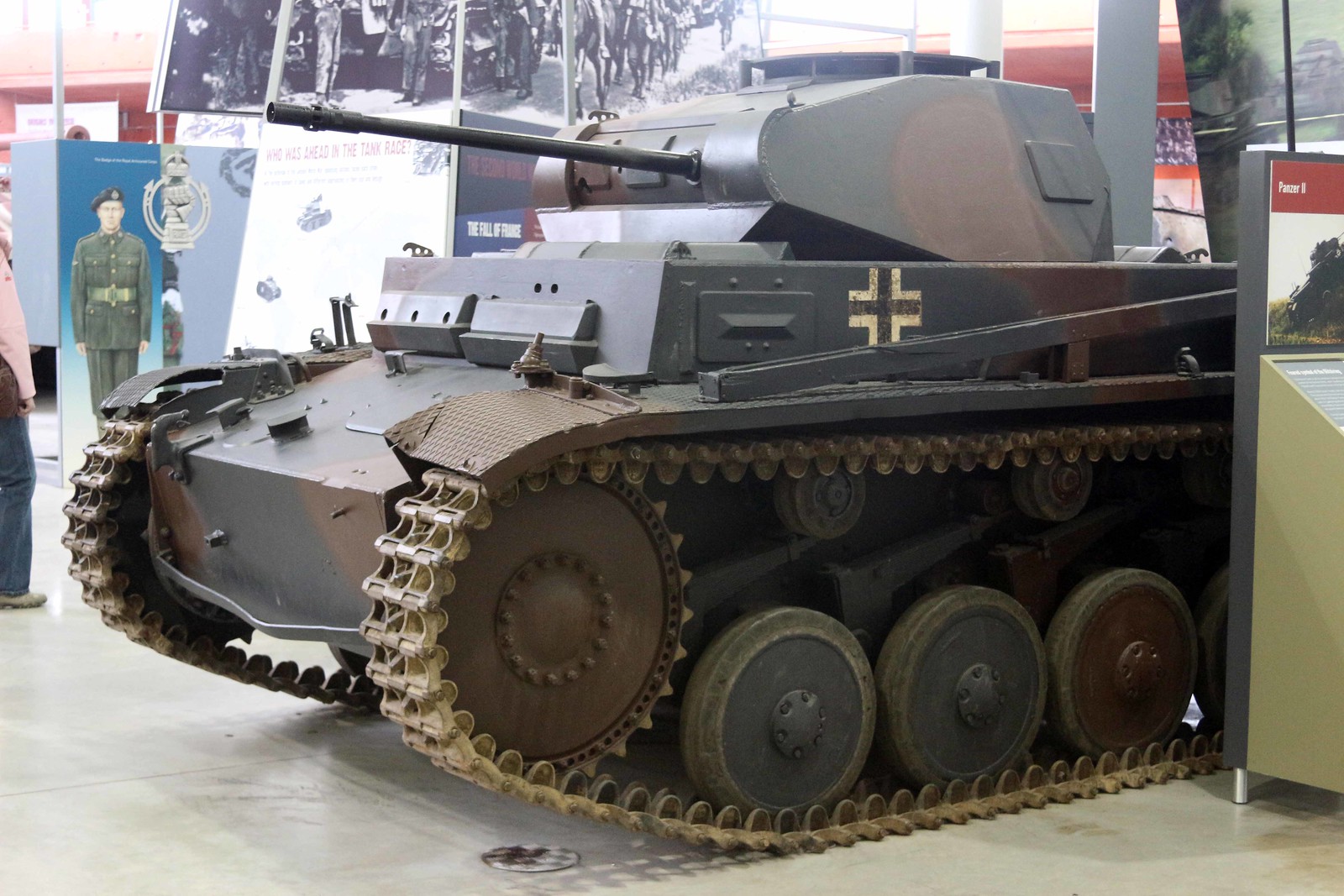This photograph, taken inside a museum, captures a detailed World War II exhibit centered around a German tank. The tank, adorned in a camouflaged mix of dark black, green, and brown colors, features a short, thin gun barrel and sports a prominent black cross outlined in white on its side. Positioned facing left, the tank's metal structure dominates the center of the image. Surrounding it are numerous black-and-white photos depicting historical scenes, some showing people riding horses while others stand next to various vehicles. A small, pole-mounted lamp fixture is also visible near the tank. 

In the background, there are more displays, including a blue wall and a red wall with a window-like feature. Adding depth to the scene, there's a color photograph of a soldier in a green uniform and beret, possibly standing as part of the exhibit. On the far left edge of the photograph, we see a partial view of a person, likely female, dressed in blue jeans and a long-sleeved pink shirt, with their hands hanging by their sides. Near the tank, there is an information kiosk, enhancing the museum's narrative of historical artifacts.